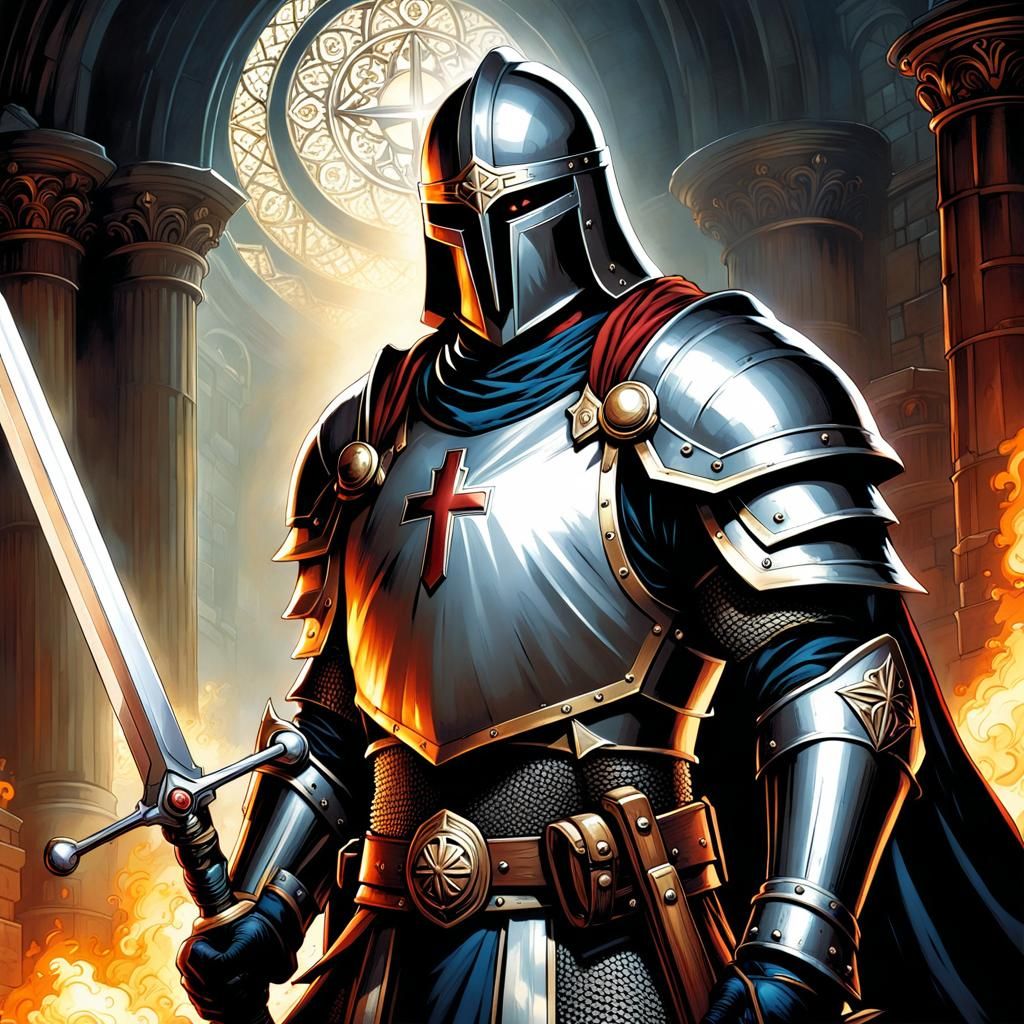In a detailed cartoon-style animated image set within a medieval church or temple, a knight in striking silver armor stands as the central focus. The background showcases grey stone walls, grand pillars, and stained glass windows through which sunlight streams, bathing the scene in a sacred light. Flames rise subtly from the ground, adding to the dramatic ambiance.

The knight, clad in shining armor adorned with gold accents, is imposing. His helmet conceals his entire face, save for a single visible, glowing left eye. A blue and red robe or cape flows behind him, enhancing his majestic presence. The chest plate of his armor features a curved design with a red crucifix prominently displayed, albeit asymmetrical and divided into three parts.

In his right hand, he wields a sword, though it appears to float just above his open palm, the hilt seemingly shorter than expected. The sword's crossguard and blade, however, are properly depicted. His attire includes a sturdy brown belt with various straps and emblems, completing his formidable appearance.